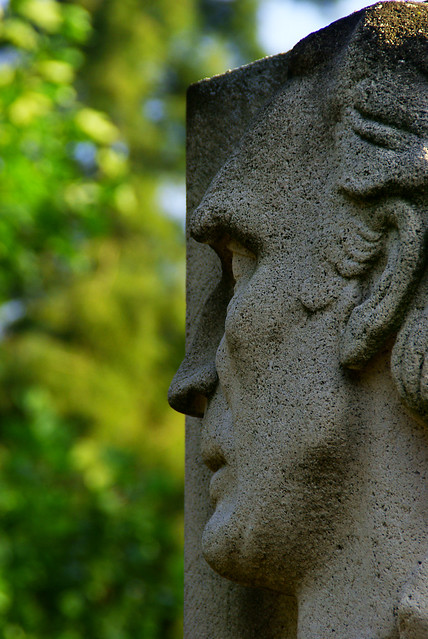The image captures a close-up view of a carved stone relief statue of a male figure, prominently featuring the left side of his face. The man, possibly middle-aged, has distinct features including deep-set eyes, a pronounced, straight Roman nose, and high, arched brows that almost hood over his eye. His ear and hair are intricately carved, with the hair extending just above and in front of the ear. The profile shows a well-defined chin and jawline, with a hint of a secondary, slightly fatty chin beneath. The statue blends into a block-like structure, which appears to have some subtle golden highlights. The stone matches the pole against which the man's head leans. Behind the statue, the background is a blur of green and yellow foliage, suggesting a sunny outdoor setting that draws focus entirely onto the intricate details of the stone carving.